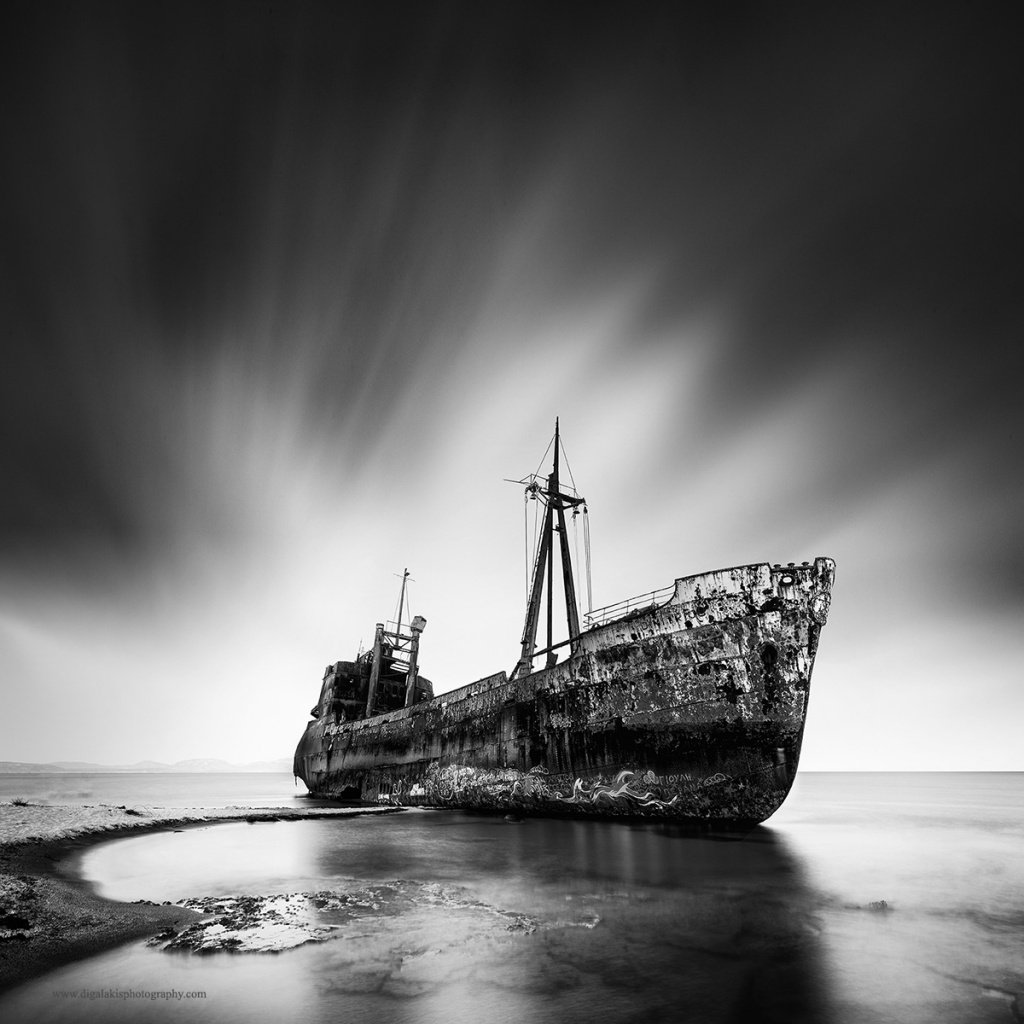A black and white photograph captures the evocative image of an old, abandoned oil tanker that appears to have run aground on a beach. From a head-on perspective, the ship's weather-beaten bow dominates the foreground, its once-white paint now marred by extensive black blotches and patches. The hull transitions to a darker shade along the bottom, interspersed with erratic white patches. Midway down the vessel, a mast rises, crisscrossed by dark lines. At the distant stern, the cabin—resembling a black box with protruding gray columns—stands in stark contrast. The ship rests on the sandy shallows of the beach, where calm, mirror-like water laps gently against the hull. The left side reveals the shoreline and hints at the beach's shallowness. The sky above is equally dramatic, starting with a white burst near the horizon that gradually deepens into a menacing dark gray as it ascends. Subtle graffiti adorns the base of the tanker, adding to its aura of neglect. In the far background, faint outlines of hills give depth to the scene, completing this poignant tableau of maritime decay.